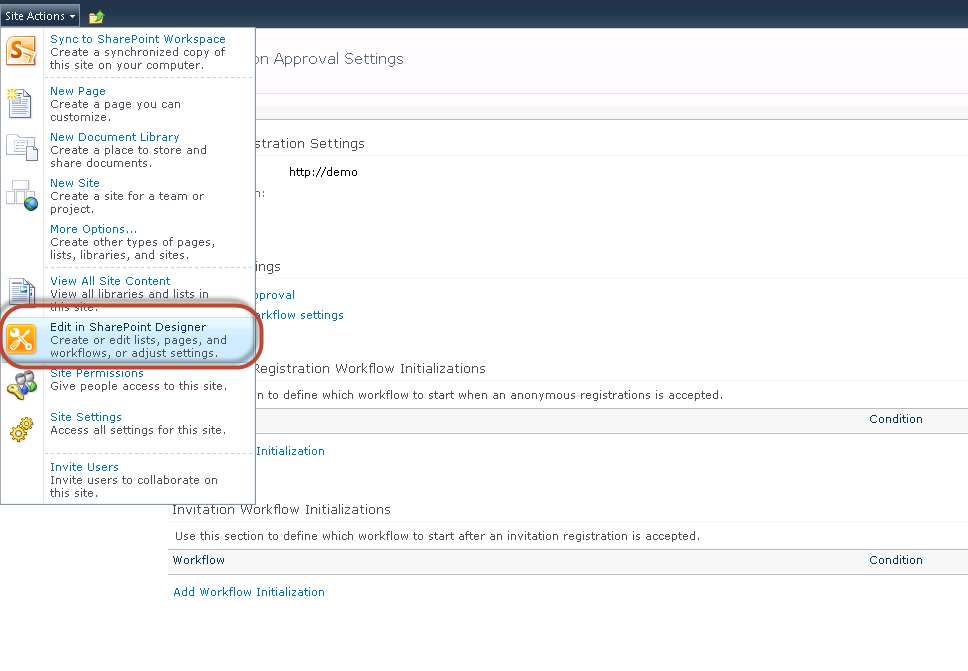The image displays a "Sites Action" screen with the title "Sites Action" prominently positioned in the upper left-hand corner within a blue bar that spans the width of the image. To the right of the title, there is a folder icon featuring an upward-pointing arrow. On the left-hand side, the image features a vertical menu with nine selectable options. The option titled "Edit in SharePoint Designer," which allows for the creation or editing of lists, pages, workflows, and settings, is circled.

This vertical menu appears to overlay another window in the background. In this background window, text related to "approval settings" and "administration settings" is partially visible, along with the URL "http://demo". Additional terms such as "condition" and "workflow" can also be seen in the background, indicating various configurations or options pertinent to SharePoint administration.